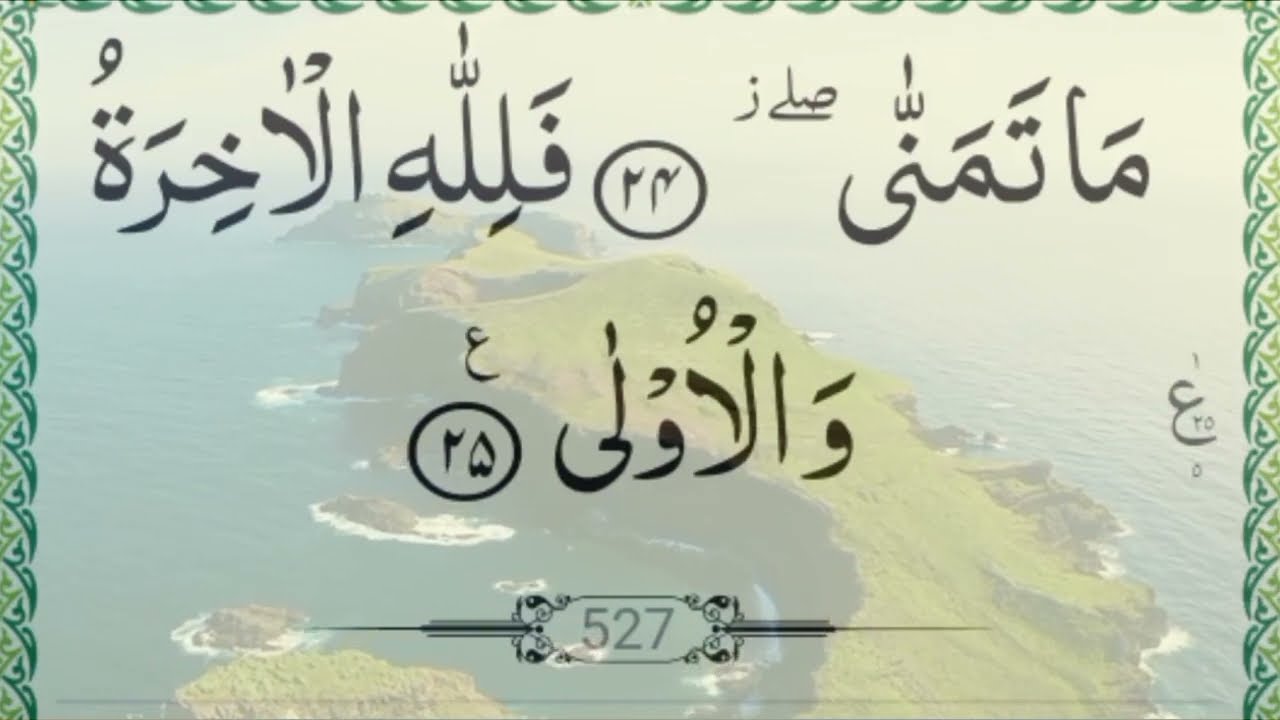The image features a green and yellow abstract background with a semi-transparent, washed-out scenery of an island surrounded by a blue-teal ocean. The island, sparsely covered in grass or shrubbery, appears like a watermark beneath the main elements. A darker green, scalloped border frames the left, right, and top edges, resembling ornamental plant-style art, but it is absent at the bottom. Dominating the top four-fifths of the image is a stylized calligraphy in an unfamiliar black script, possibly Arabic. Centrally positioned at the bottom is an oval containing the number 527, flanked by small clamp-like symbols that extend horizontally from either side. Additionally, there are two circles with individual characters within them, interspersed with random notes scattered across the image.